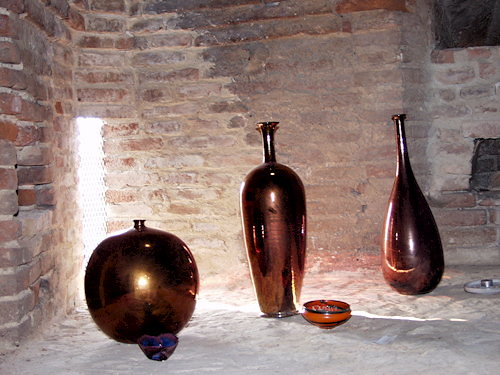This high-quality color photograph captures three distinctive brown brass vases and two shorter ceramic bowls against a dusty, brick red background with a sandy, rough floor. The scene appears to be inside an old, possibly re-mortared, brick building with a section of bright sunlight streaming through a narrow rectangular window on the left.

The vase on the left has a short, almost apple-shaped body. In front of it sits a small, blue and black ceramic bowl. The central vase is taller with a wide, oblong body tapering to a skinny neck. In front of this vase is an orange and black bowl. The third vase on the far right has a teardrop shape with a rounded bottom that narrows to a long, slender neck. A white lid or plate is placed on the ground next to this vase. All three vases display a shiny surface that reflects light, adding a luminous quality to the image.